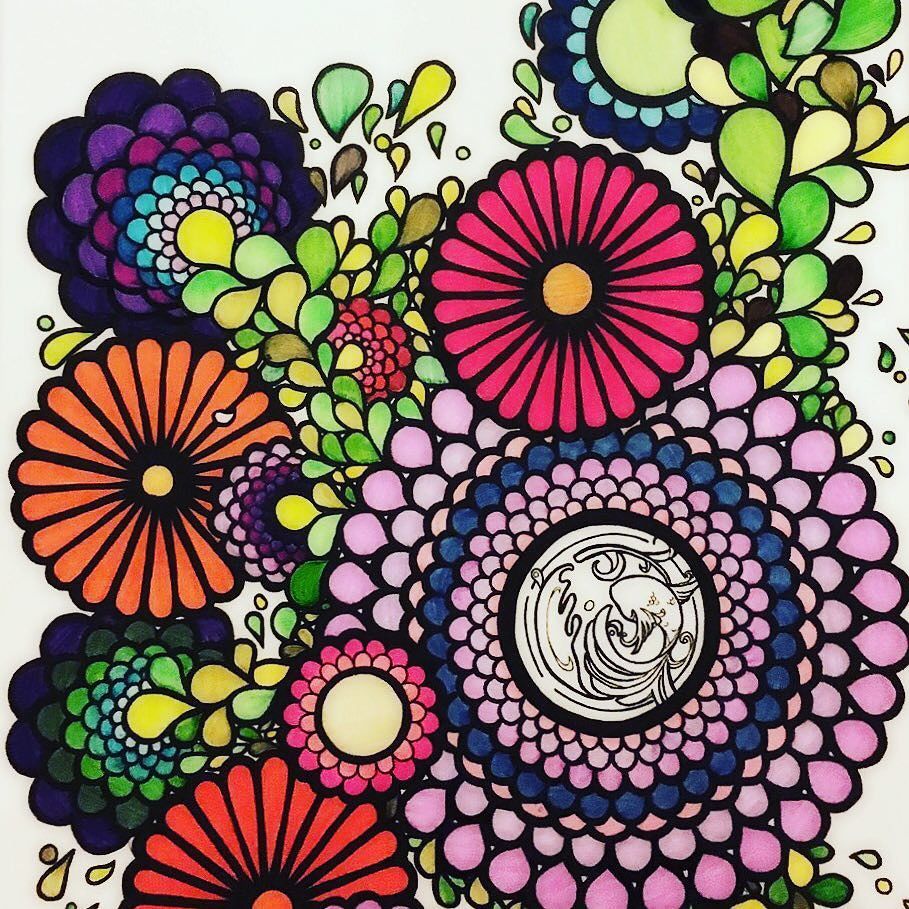This vibrant and intricate image features a mesmerizing array of colorful circular and teardrop-shaped designs. At the bottom center, there is an orange circular shape resembling a sunflower. Above it, to the left, is a series of circular elements in shades of blue, green, and yellow. To the right of these, a captivating circular design combines purple and pink with a white center. Dominating the composition is a grand purple structure, which contains an inner blue ring, a black ring, and white designs at the core. Scattered throughout are smaller teardrop-shaped objects in light green and yellow hues. A pink sunflower outlined in black with a yellow center adds to the visual feast. In the top left, a striking flower-like pattern emerges, comprised of dark purple, light purple, pink, blue, and white segments. The overall composition is set against a pristine white background, emphasizing the vividness of the colors and the complexity of the design.